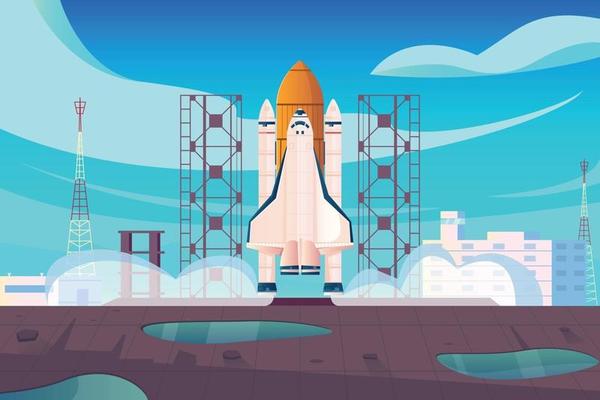The image depicts a meticulously designed graphic representation of a space shuttle launch site. Dominating the center is a sleek, white spaceship adorned with blue-tinted edges on its wings and blue windows. Flanking the spaceship are two similarly colored boosters, all anchored to a taller, commanding orange rocket in the background. On either side of the rocket assembly, large metallic structures tower, likely serving as access points for personnel to board the spacecraft. 

To the right of the scene, a prominent white building stands alongside two towering structures that resemble radio towers. On the left, smaller white buildings are scattered across the landscape. The ground below is a rugged brownish-red terrain, sporadically marked with greenish puddles.

The sky above transitions from a deep blue at the zenith to a greenish hue closer to the horizon, accentuated with stylized, swirling clouds. Beneath the rocket, wisps of smoke artistically billow, adding a dynamic feel to the image.